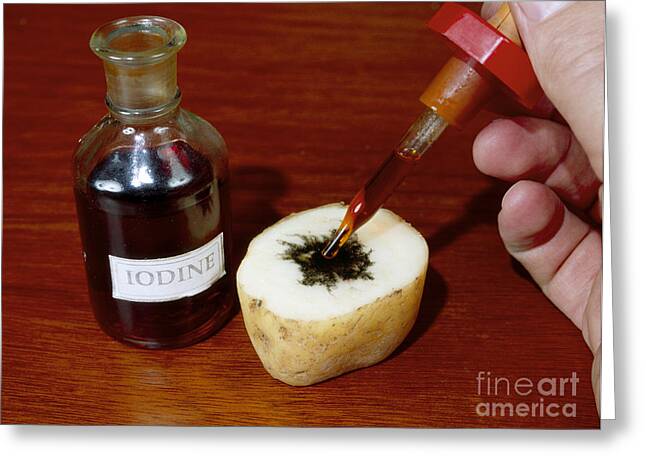In the center of the photograph, there's a small, nearly half-filled glass vial with a white rectangular label that reads "IODINE" in gray, all capital letters. It sits on a dark wooden table or countertop that forms the background of the image. To the right of the vial lies a freshly cut potato slice, with its brown skin on the side and the white, flat, peeled edge facing upwards. A person’s fingers, visible on the far right, holds a dropper filled with a reddish-brown liquid, presumably iodine. The dropper releases a drop of the iodine onto the white part of the potato, creating a blackish spot upon contact. In the lower right-hand corner of the image, the text "Fine Art America" can be seen.